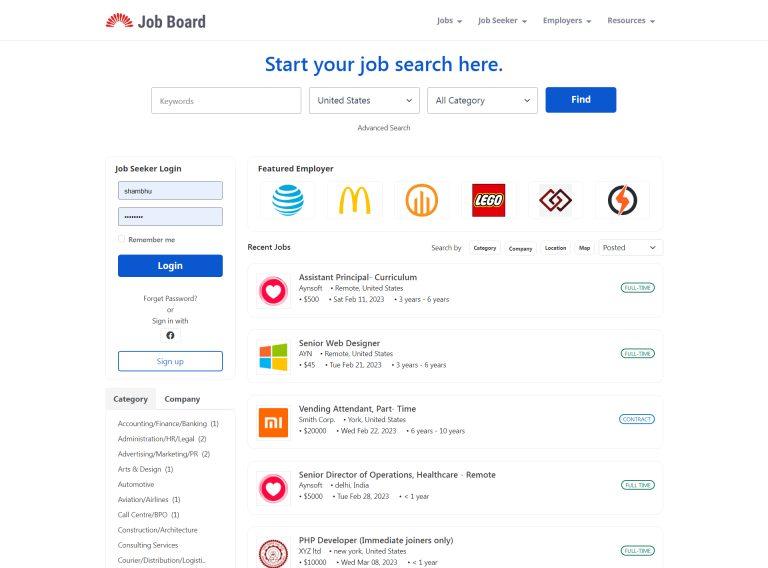This is a cropped screenshot of a job board web page. At the top left of the page, the job board logo is prominently displayed. On the right side of the page's header, there are four categories with drop-down boxes labeled "Jobs," "Job Seeker," "Employers," and "Resources." Directly beneath the header, the phrase "Start Your Job Search Here" is centered on the page in bold blue letters. Below this heading, there is a keyword text box, accompanied by a drop-down box set to "United States," another drop-down box set to "All Categories," and a blue "Find" button.

On the left side of the page, a panel is titled "Job Seeker Login" at the top. This section includes fields for entering a username and password, along with a large blue "Login" button. Additional options below this include "Forgot password?" and "Sign in with Facebook." Further down the left column, the panel displays "Sign Up," followed by headings "Category" and "Company" with a vertical list of categories beneath the "Category" heading.

On the right side of the panel, the top section highlights "Featured Employers," showcasing a horizontal list of company logos including AT&T, McDonald's, and Lego. Below this, the phrase "Recent Jobs" appears in small letters toward the left side, accompanied by a vertical listing of recent job postings.

Overall, the layout is designed to facilitate easy navigation and efficient job searches, with clear sections for job seekers to log in, sign up, and find openings from featured employers.